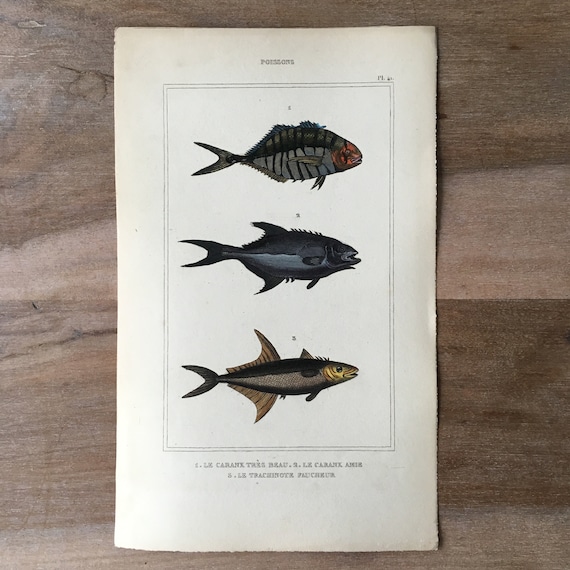The image captures a color photograph of what appears to be a page from a book or a magazine, featuring illustrations of three different fish, all facing towards the right. The page, which is white with a double black border, is positioned on a brown wooden tabletop. Each fish is numbered from 1 to 3 and spaced equally apart. The top fish is medium-bodied with a gray hue and brown accents. The second fish in the middle is also medium-bodied and predominantly gray. The third and smallest fish at the bottom has large fins and is adorned in black and green or yellow-green colors. The text on the page, although blurry and difficult to decipher, includes explanatory notes at both the top and bottom, with the bottom text containing the names of the fish. The photograph is taken from above, giving a clear view of the entire page against the wooden background.